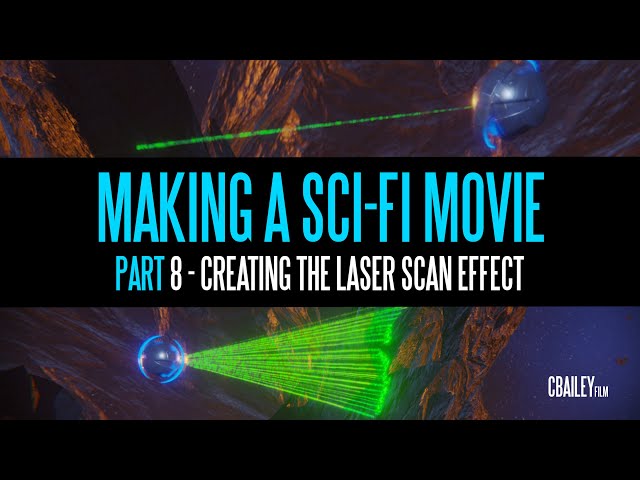The image is a detailed movie poster for a sci-fi film. At the center of the poster, large text in dark and light blue, all caps font reads: "MAKING A SCI-FI MOVIE." Directly below this, in smaller white font, it states: "PART EIGHT: CREATING THE LASER SKIN EFFECT." At the top and bottom of this central text, two thick black lines span the width of the poster.

Above the top black line, there is a scene showing a small gray ball emerging from a darker gray rock, emitting a green laser beam towards the left. Below the bottom black line, within a swath of gray sky, another scene depicts a blue, gray, and purplish ball. This ball, not lodged into the rock, is shooting multiple green lasers to the right. Surrounding this scene, near the top left, a bluish-purple sky dotted with white stars creates a cosmic backdrop.

To the bottom right of the image, white text reads: "SEE BAILEY FILM." The overall color scheme combines shades of blue, gray, green, and purple, accentuating the sci-fi theme of laser beams and cosmic elements.